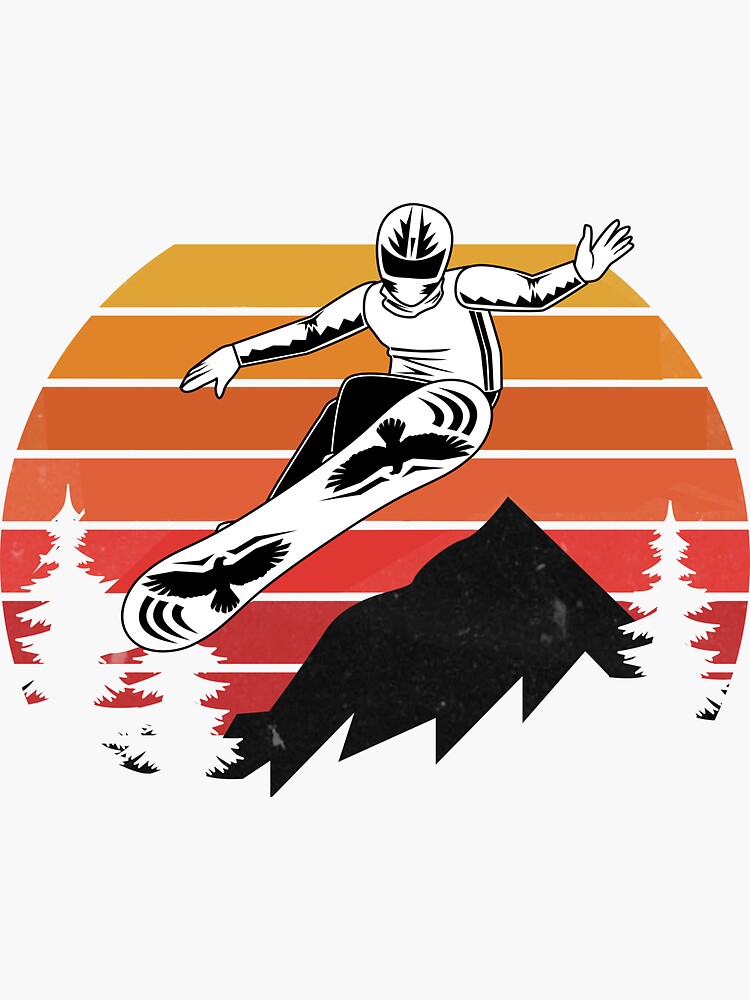The image depicts a stylized, digital illustration of a snowboarder caught mid-jump against a white background. The snowboarder, primarily rendered in white with black details for shadows and accents, sports a helmet adorned with small, pointed designs and a black visor. His attire includes a white shirt with black triangular spikes on the sleeves and black pants. Notably, the snowboard's underside showcases two black silhouettes of birds with outstretched wings, positioned alongside lion-like figures. The scene behind the snowboarder features a black mountain silhouette, white trees, and a striking horizon. The sky transitions from a yellow top to a reddish bottom, segmented by lines that give it a striped appearance, suggesting either a sunset or sunrise. The entire composition is framed with elements reminiscent of a wooden panel backdrop in shades of yellow, orange, and red, enhancing the dramatic and energetic atmosphere.